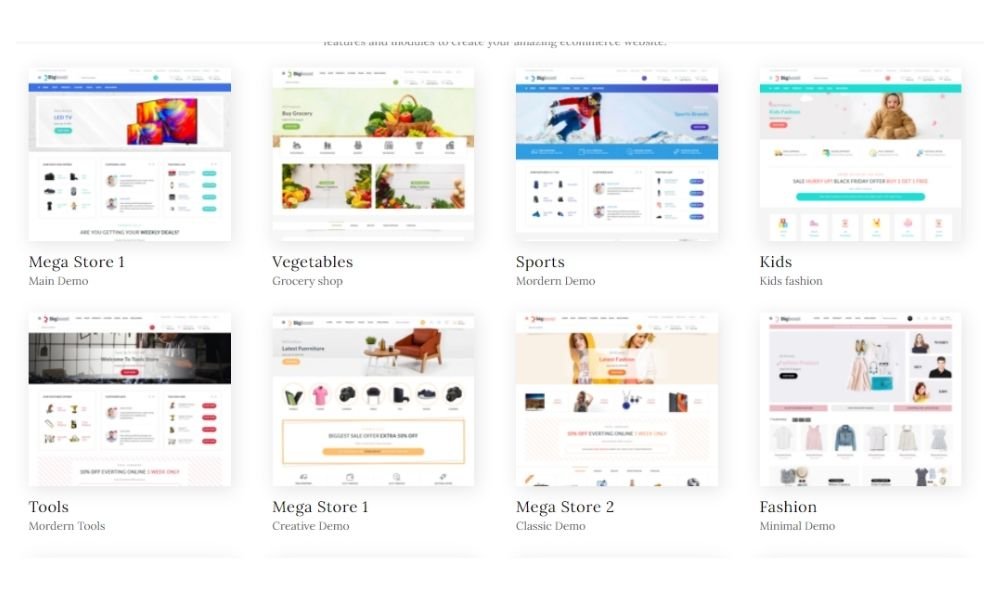Screenshot of a website displaying eight demo site examples, showcasing the diverse range of templates available. The background is predominantly white, and the demos are organized into two rows of four. 

- **Top Left: "Megastore 1 Main Demo"** - Features a clean layout with multiple product images against a white background.
- **Top Center Left: "Vegetables Grocery Shop"** - Displays vibrant produce in the background with icons representing different shopping categories.
- **Top Center Right: "Sports Modern Demo"** - Captures the dynamic action of a skier front and center.
- **Top Right: "Kids and Kids Fashion"** - Showcases an adorable child dressed in a brown, furry suit.

- **Bottom Left: "Tools Modern Tools"** - Highlights a practical workshop setting.
- **Bottom Center Left: "Megastore 1 Creative Demo"** - Features elegant furniture in a stylish, modern layout.
- **Bottom Center Right: "Megastore 2 Classic Demo"** - Presents two women in fashionable attire, set against a peach-colored background.
- **Bottom Right: "Fashion Minimal Demo"** - Displays a minimalist design highlighting various clothing products.

Each demo site offers a unique design theme, catering to different types of businesses and aesthetics, akin to a service like Squarespace.